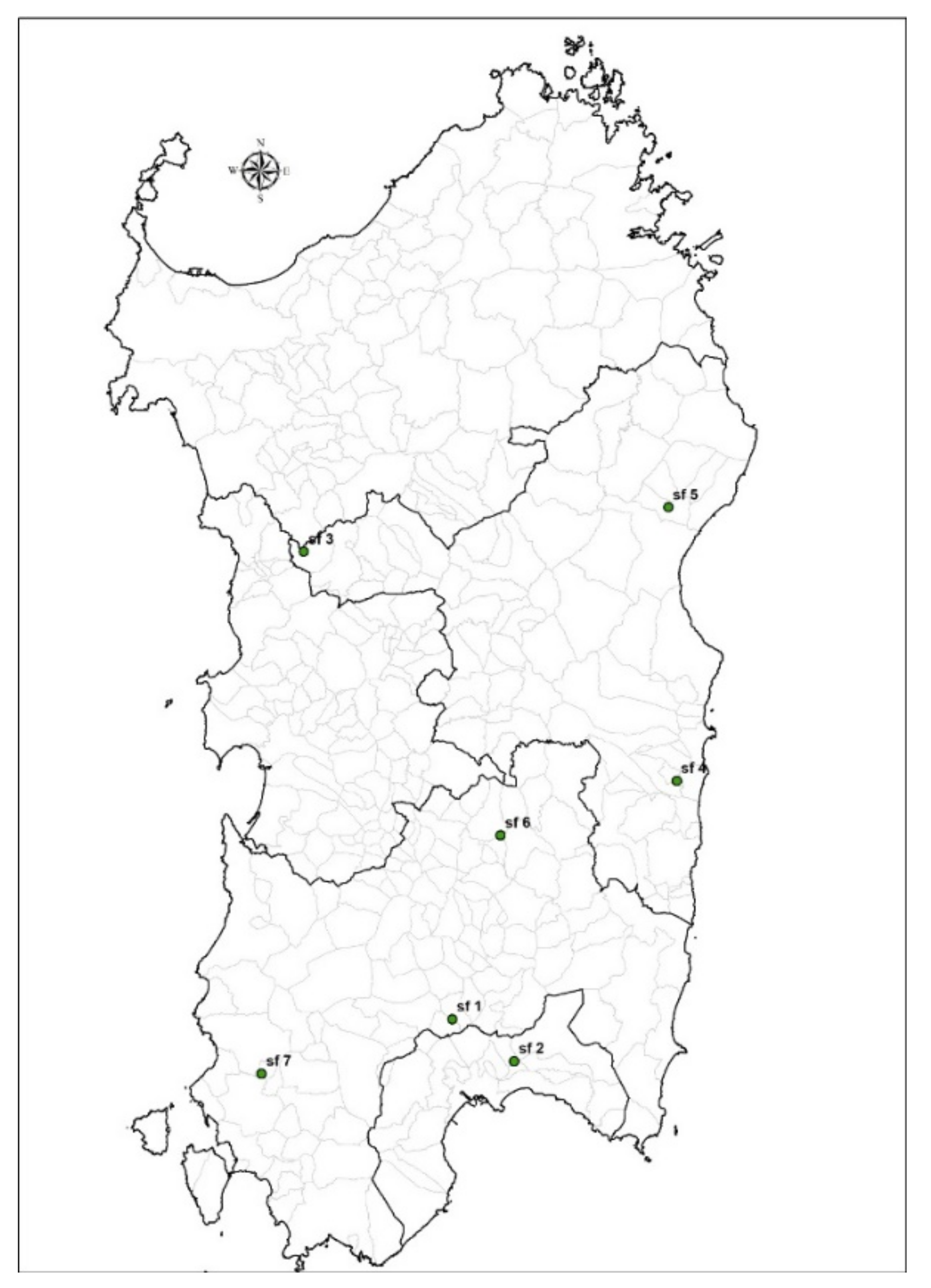This is a detailed black-and-white map of Sardinia, rendered in a line drawing style and divided into five main sections. The sections are further sub-divided into smaller areas resembling counties or cities. A compass indicating the cardinal directions is positioned at the top left corner. Notably, the map features seven small green dots labeled SF1 through SF7, which are the only elements of color. These green dots are scattered across the map, with some sections containing more than one dot and others having none. The map does not include any legends, water bodies, landmarks, or names of cities and capitals, leaving the significance of the green dots ambiguous. The overall shape of the map is rough, vertical, and rectangular, with the smallest section at the bottom and the largest at the top.